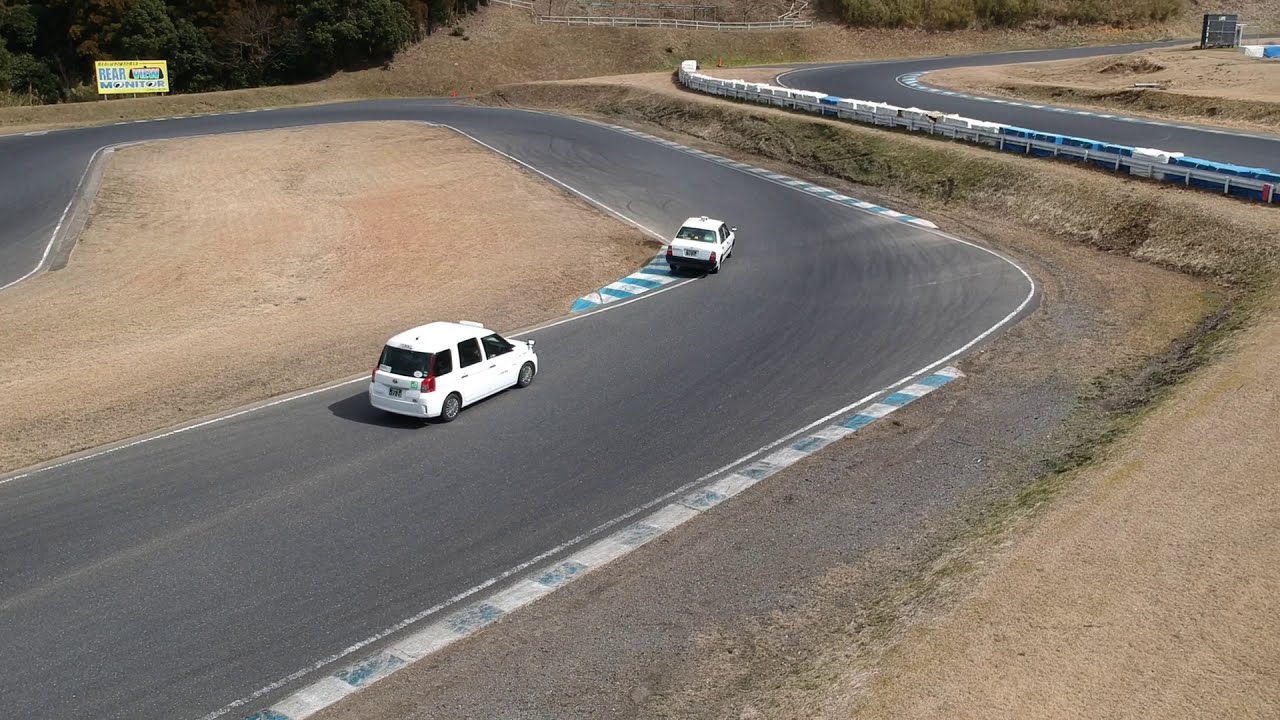This photograph captures a dynamic scene of two white cars navigating a complex, paved gray racetrack that twists and turns through a light brown dirt landscape. The track features various contours, including a higher elevated section visible in the upper right corner of the image. Around the track, brown dirt banks act as barriers to absorb any potential off-road incidents, providing some safety measures. 

Within the infield of the track, a flat, dirt area contrasts with the more built-up banks on the outside. The two white cars, appearing to be a four-door sedan and a four-door hatchback, are racing closely. The sedan is positioned slightly above the center of the image, while the hatchback is trailing slightly down and to the left. Adding to the scene's detail, one of the cars is seen cutting through a blue and white striped separator on an inner corner, seemingly taking a shortcut.

A yellow rectangular sign with partially legible blue lettering, situated in the upper left corner, adds a splash of color to the otherwise neutral-toned environment. Additionally, a fence topped with barricades runs along the upper section of the track, acting as a safety barrier. The photograph is taken from a slight elevation, possibly a dirt ramp, providing a broad view of the racetrack without showing any spectator bleachers.